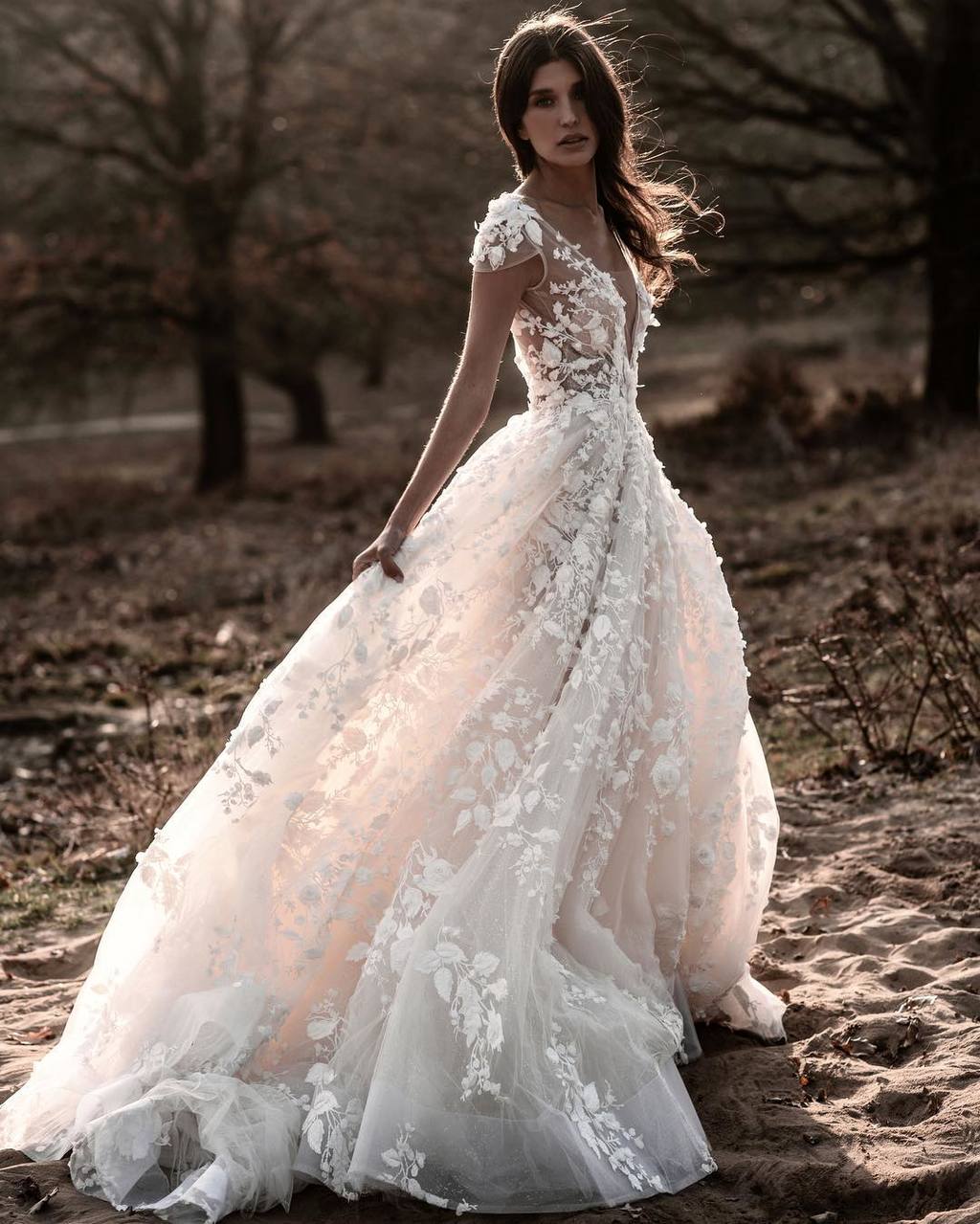The image depicts a striking piece of fashion photography featuring a young woman standing gracefully on a sandy expanse, likely a beach. She is wearing an elegant wedding dress that highlights her natural beauty. The dress is intricately designed with a floral pattern woven into the lacy, translucent fabric. The gown, which is low-cut in the front, cascades down in a long, flowing skirt that billows in the wind. The ethereal effect of the semi-transparent dress is heightened by the glowing backlight from the sun, illuminating her skin and the exquisite floral embroidery. Her long, dark hair, which falls below her shoulders in wavy, flowing locks, is gently lifted by the breeze, adding to the cinematic quality of the scene. She holds the back of her dress with one hand, striking a poised and dramatic pose as she gazes into the camera. The background features a mix of sandy terrain and a forested area with trees, some of which are devoid of leaves, suggesting a fall setting. The interplay of natural light and fine fabric details amidst the serene outdoor setting makes this image a captivating piece of fashion photography.